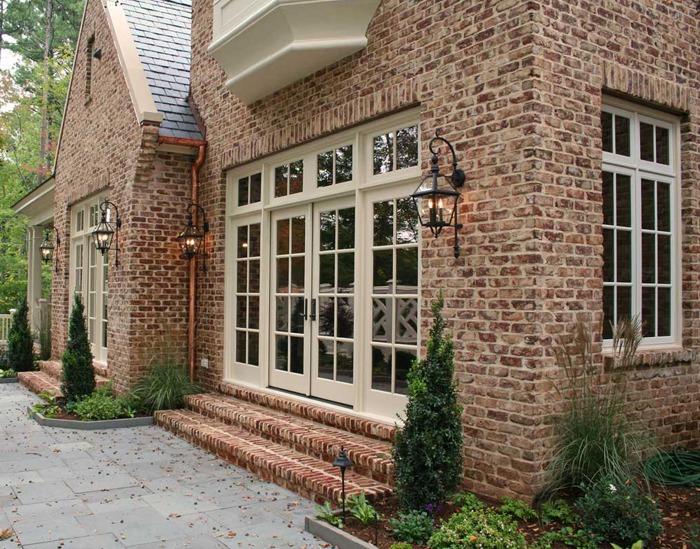This photograph depicts an elaborate, well-maintained brick mansion with bricks in varying shades of red, orange, beige, and brown. The central focus is on the French doors, which are glass-fronted and white, framed by two steps and flanked by wrought iron lanterns that are lit, adding an old-style charm. Surrounding the entrance are small evergreen shrubs and further shrubbery to the right and left. 

Above the entrance, four windows line the facade, and adjacent to the door, we observe another section of the building with a window featuring white panes. On the left side, more windows lead to a covered front porch supported by large white pillars. A large tree with a canopy of green leaves, transitioning to yellowish-green near the bottom, cascades over the house. The roof, made of gray slate or standard tiles, is complemented by bronze gutters and beige spouting.

In front of the entrance, a grey stone pathway made of flagstones extends towards the foreground, flanked by mulch in the garden areas. The photograph, taken during the day, reveals a backdrop of tall trees, enhancing the picturesque setting of this grand single-family home.